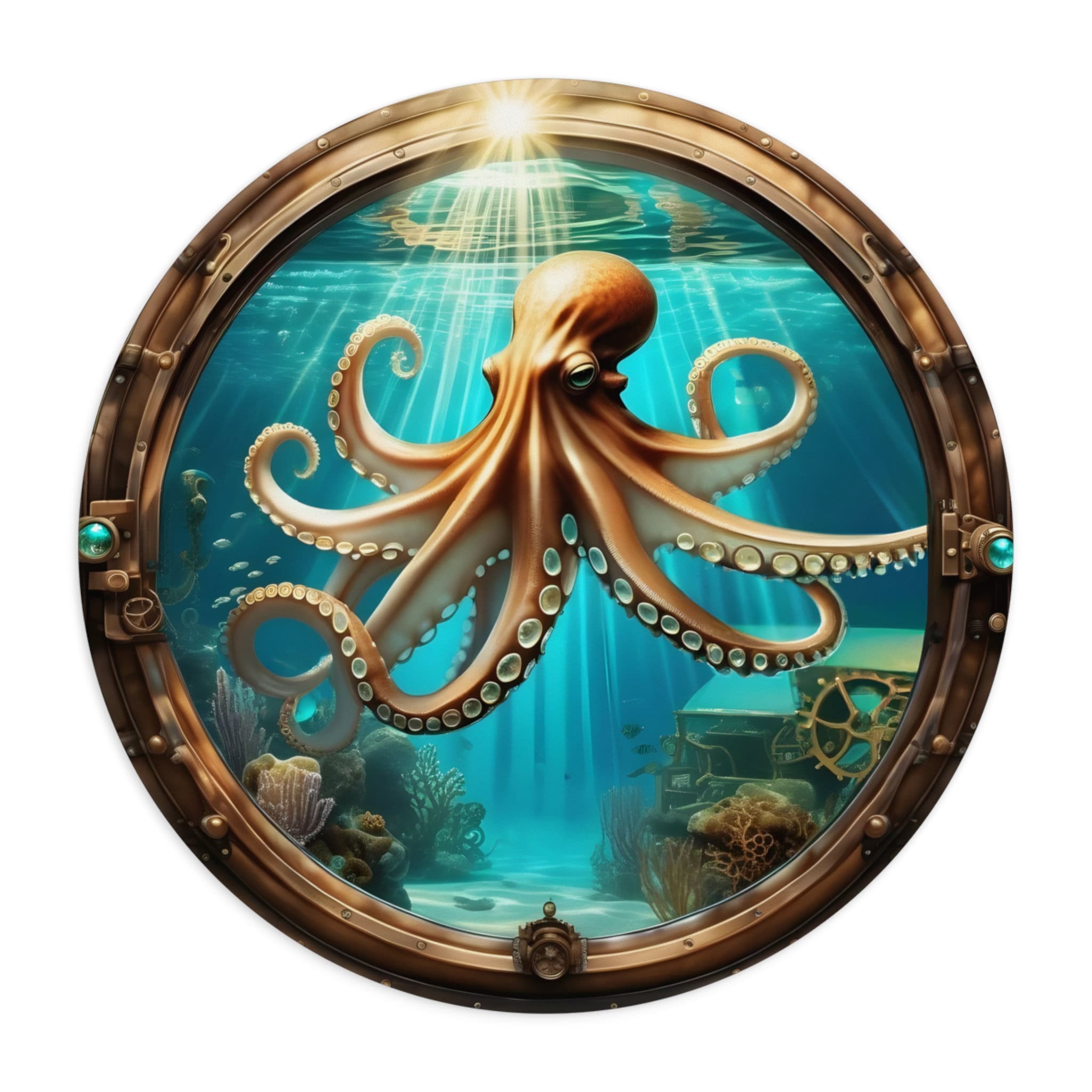The image depicts an underwater scene viewed through a thick, gold-rimmed porthole, resembling one found on a submarine or a ship. Central to this view is a striking octopus, predominantly light brown with touches of orange, exhibiting a large head and flared, curling tentacles adorned with distinctive white suction cups. The background is an ocean tableau lit by beams of sunlight filtering down from the shimmering surface above, casting a mesmerizing glow on the scene. The ocean floor features sand, vibrant coral reefs, seaweeds, and additional marine life, including small fish. Additionally, an abandoned green machine with a gold gearwheel adds an element of intrigue to the scene. The porthole itself is set against an all-white background, accented by small, blue-knobbed adjustments on either side, enhancing the impression of a sturdy maritime window.